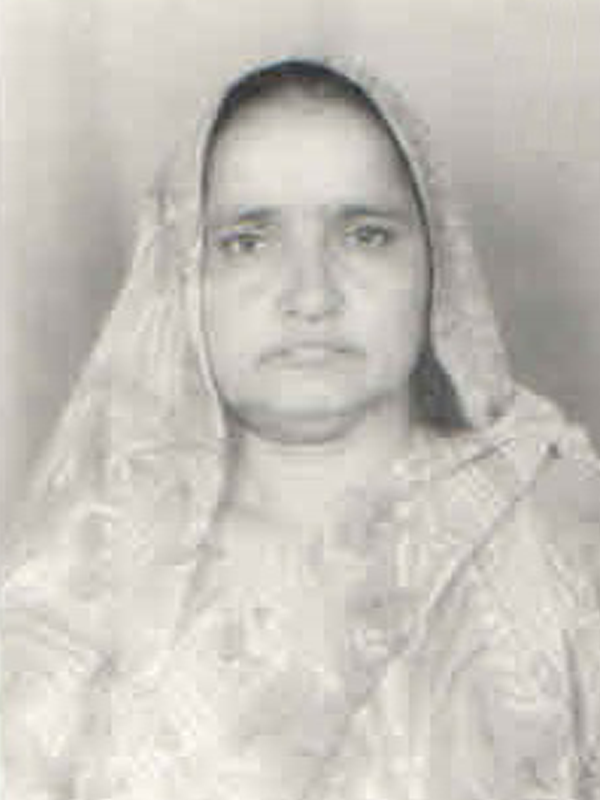This hazy, highly compressed, black-and-white photo depicts a woman clad in what appears to be an ornate religious robe that fully envelops her body, featuring a hood that covers her head. Despite the severe JPEG artifacting and overall blurriness that obscures finer details, subtle patterns can be discerned throughout the robe. Her hair, or possibly shadows beneath the hood, appears dark, and her eyes seem to be a light color, perhaps blue or gray, though the resolution makes it hard to confirm. The woman, possibly of Middle Eastern descent, has a grim and somber expression, with her lips drawn downwards. The photo's indoor setting with a white backdrop adds to the bleak and gloomy atmosphere conveyed by the image.